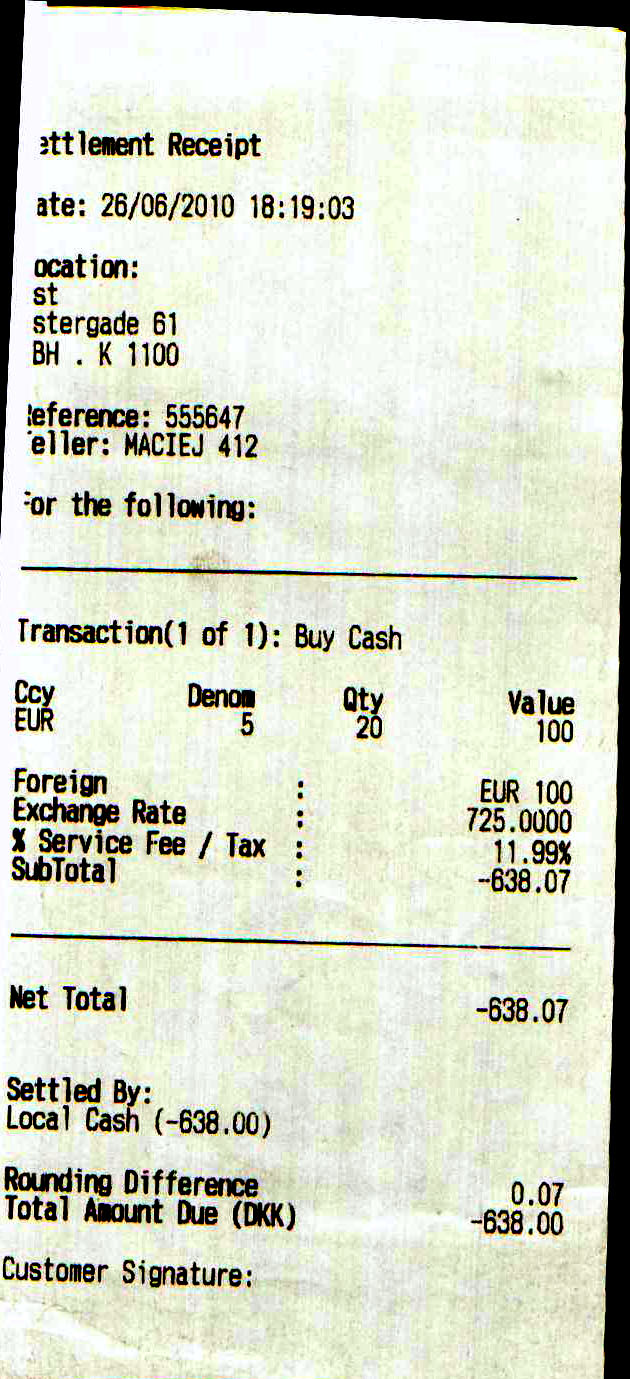The image displays a printed paper receipt titled 'Settlement Receipt' dated 26-06-2010 at 18:19:03. The top and left margins are partially cut off, and the location details are not fully legible. It references number 555-647 and the teller identified as "Macay 412." Below a black dividing line, it indicates: "Transaction one of one by cash." The receipt details multiple columns: 

- "CCY" (currency: Euro)
- "Denom" (denomination: 5)
- "Qty" (quantity: 20)
- "Value" (100)

The receipt further outlines a foreign Euro value of 100, an exchange rate of 7.25%, and a service fee/tax of 11.99%. The subtotal and net total both read as -638.07, settled by local cash amounting to -638 with a rounding difference of 0.07. The final amount due is listed as DKK -638. The section for the customer signature is present but remains unsigned.